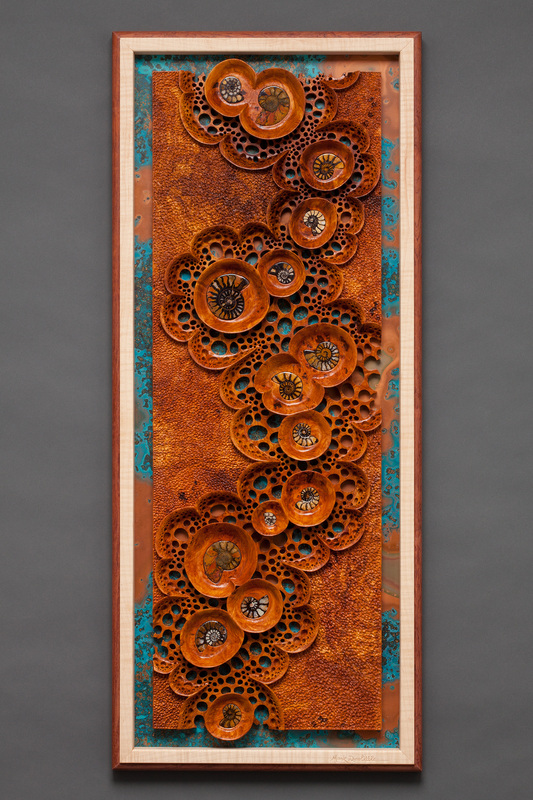This image depicts a vertically oriented, framed modern art piece hanging on a dark slate-gray wall. The frame itself is burnt orange with a white inner border, adding a layered depth to the presentation. The artwork features an abstraction primarily in shades of orange, comprising overlapping circular forms that evoke the intricate, organic structure of mushrooms or fungus. The background contrasts with these warm tones, showcasing hues of teal, seafoam blue, and black with a splattered effect. The circles with various designs are arranged in a sinuous, snake-like pattern, enhancing the dynamic composition. This intricate and decorative piece of art appears designed for visual interest rather than depicting a specific subject, making it a fitting installation in a museum of modern art.